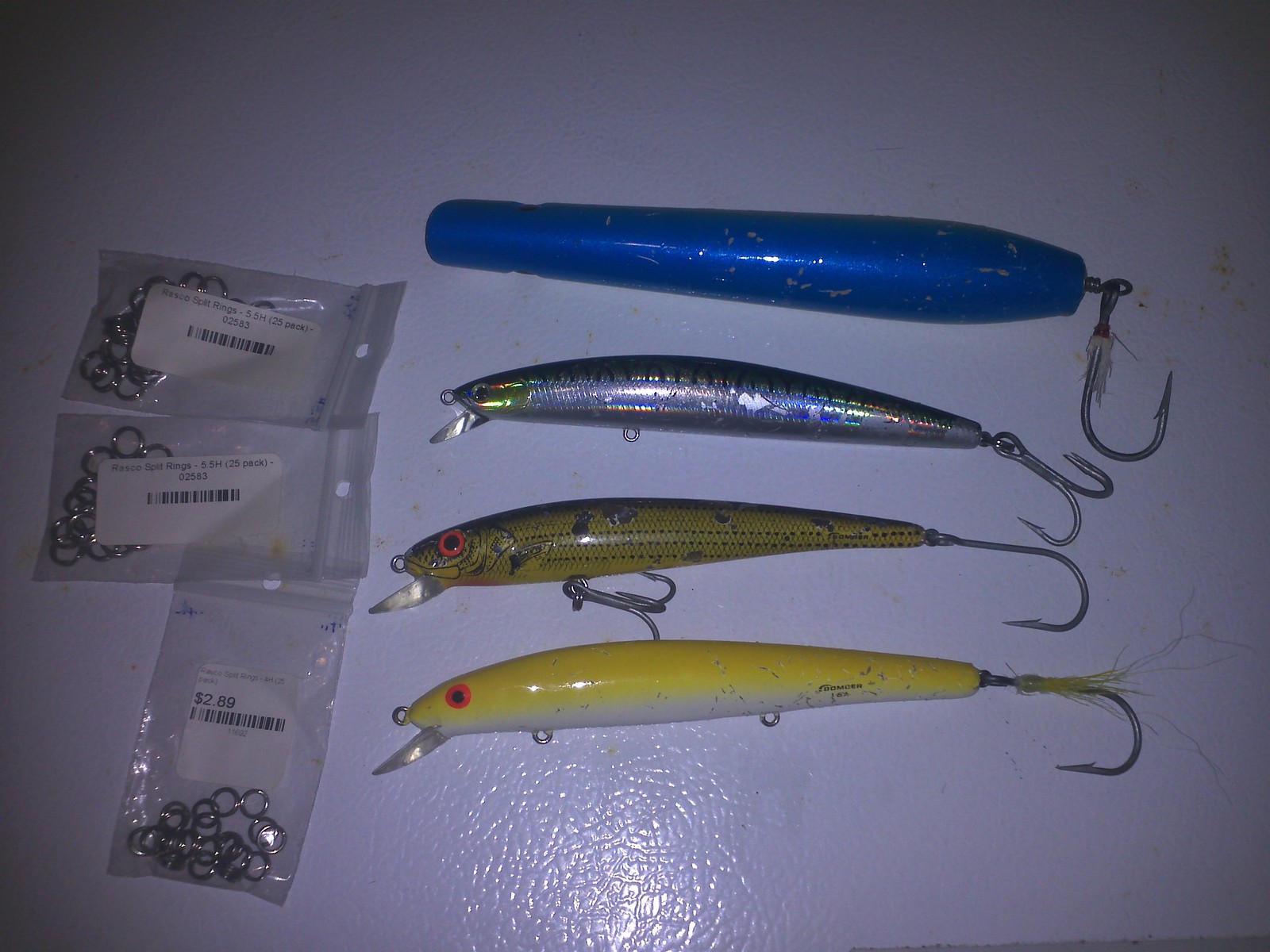The image showcases a close-up photograph of fishing lures and equipment displayed on a white countertop under bright indoor lighting, which accentuates the vivid details of the lures. On the right side of the photograph, four distinct fishing lures are aligned in a row. The topmost lure is dark blue with light gray specks, featuring a large single hook. The second lure is silver, with a green reflective tip and a treble hook, mimicking a fish with pronounced eyes—gold with black pupils. Next is an olive green lure with black stripes and red eyes, sporting a single hook. The bottom lure is yellow and white, adorned with dark brown markings from use, an orange eye with a black center, and a small knife-like shape at the front. 

To the left, three small Ziploc bags containing eye hooks or silver rings are neatly laid out, each with labels and ISBN codes. The white countertop highlights the organized arrangement and intricate details of the fishing gear, creating a vivid and comprehensive representation of the equipment.